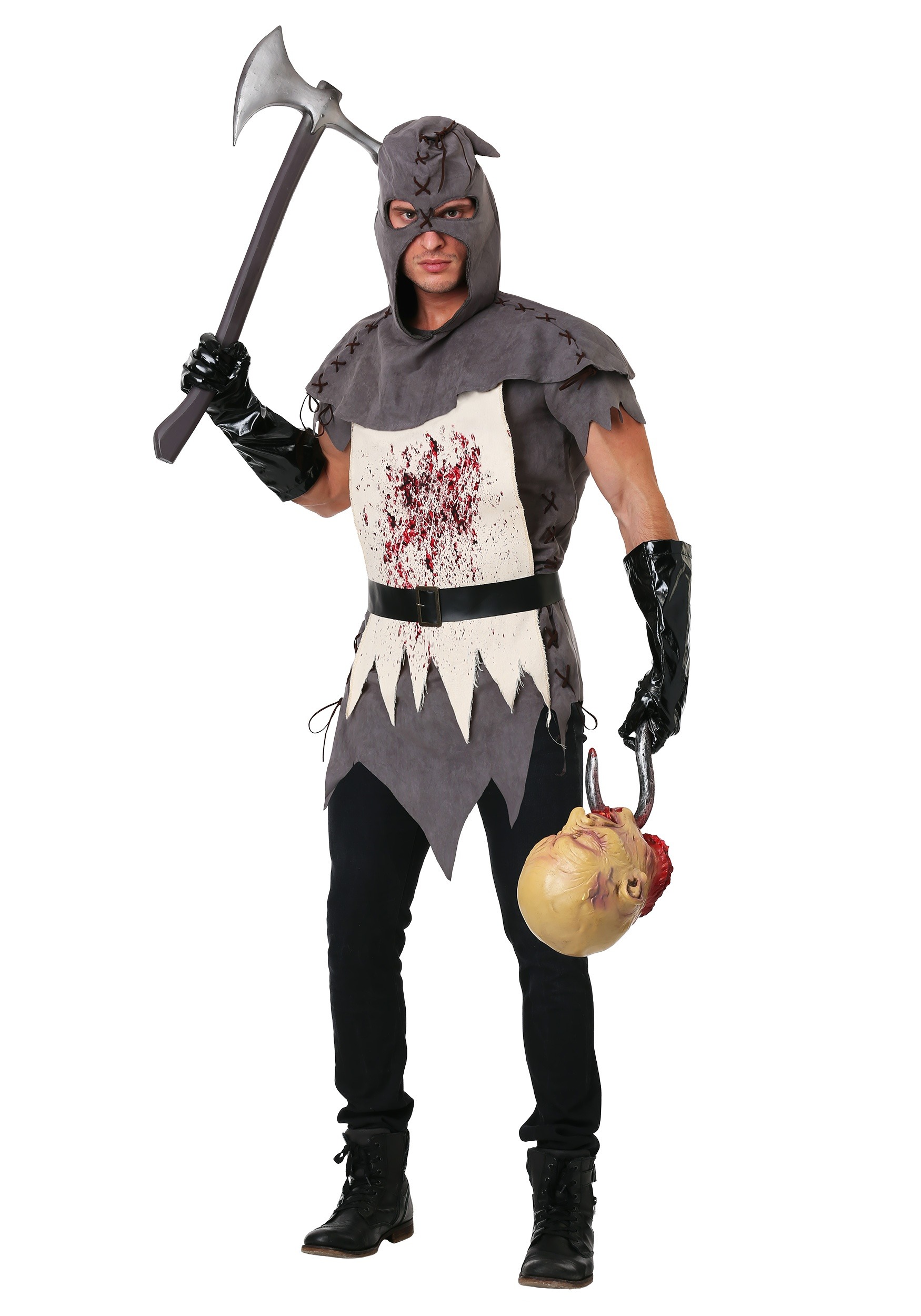The image features a Caucasian man dressed in a medieval-style executioner's costume, demonstrating a detailed and somewhat grim ensemble. The costume consists of a gray hood that covers his forehead and extends down to expose only his eyes, nose, and mouth. This hood is attached to a gray, tattered cloak-like tunic with jagged edges, suggestive of coarse materials like leather and linen. The tunic ends below his waist and is complemented by a black belt that secures a white apron-like panel at the front, stained with splatters of fake blood in dark red and black hues.

The man is also wearing shiny black leather gloves, black pants, and black boots, adding to the dark, foreboding nature of his attire. In his right hand, he wields a stylized axe with a black handle, while his left hand grips a hook that gruesomely suspends a fake severed head, with the hook piercing under the chin and exiting through the mouth. The executioner poses with an intense stare directed at the camera, taking the photo with serious and eerie intent.